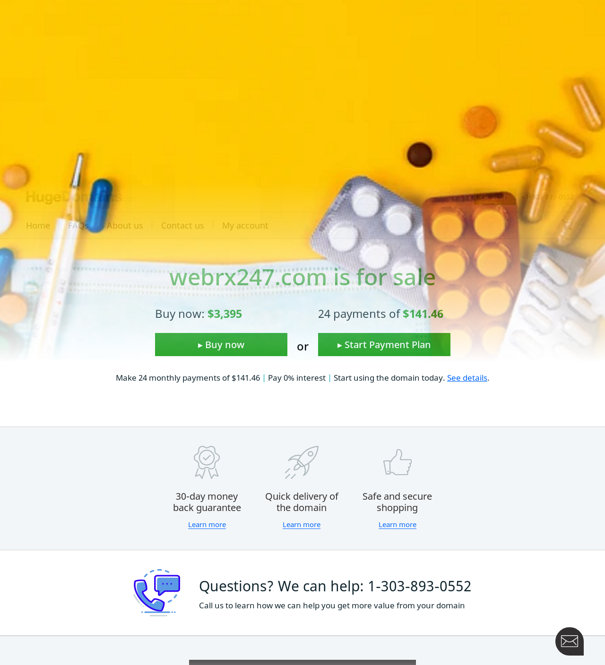The image is a screenshot of a webpage from WebRx247.com, which is currently for sale. The webpage has a light orange-yellow background that contrasts with the prominent text. At the top, in bold green letters, it states, "WebRx247.com is for sale." 

On the right side of the image, there is an assortment of medication: six capsules and two loose pills, along with several packets of pills. These packets hold pills that can be pressed out, with one packet containing white pills and the other containing orange pills.

On the left side of the screenshot, there is a blue capsule and an orange-yellow pill, alongside a slender silver object that resembles either a pen or a thermometer.

Below the announcement about the website being for sale, there's a pricing section. It states "Buy it now" at a price of $3,395, accompanied by a green "buy now" button. There's also an alternative payment option of 24 installments at $141.46 per month, with an adjacent green button labeled "start payment plan."

Further down, there's a wide light gray bar featuring three icons: a prize, a rocket ship, and a thumbs up. These icons are accompanied by text that reads "Money Back Guarantee," "Quick Delivery of the Domain," and "Safe and Secure Shopping."

At the bottom, there's a section labeled "Questions" with an icon of a telephone, indicating a point of contact for inquiries.